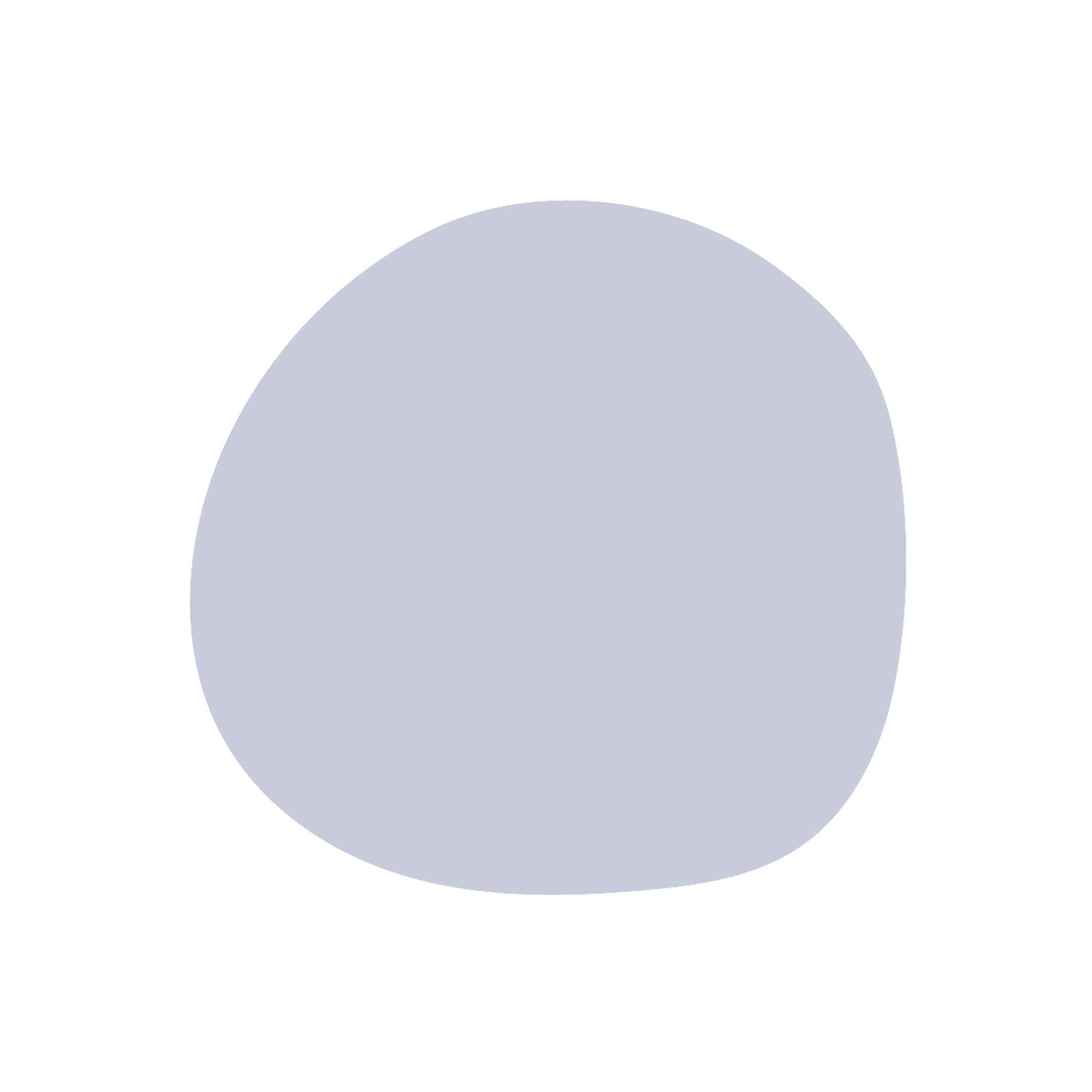The image depicts a modern art piece showcasing a pale lavender-blue blob against a stark white background. The blob, which has an irregular, almost circular shape, resembles a boulder or a rounded mass. Its surface is a solid, muted grayish-purple, without any shading or light dynamics. This simple, nondescript object is centrally positioned on the plain white canvas, suggesting it might be a digital rendering rather than a photograph, possibly created with a basic drawing tool like Microsoft Paint. Despite its unassuming appearance and lack of distinctive features, the artwork evokes a minimalist aesthetic.